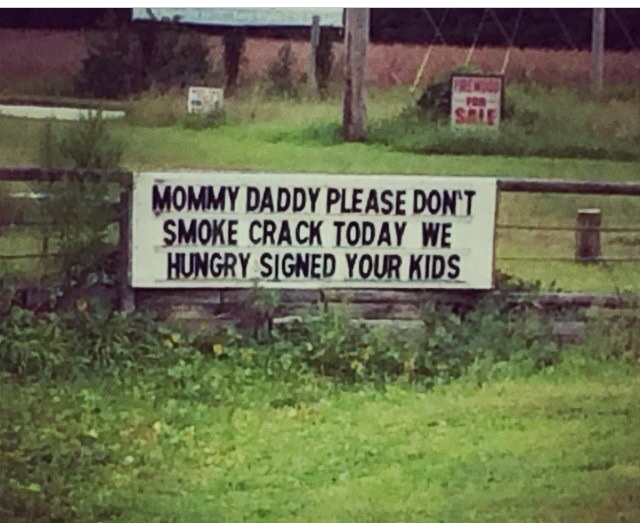In this detailed, possibly filtered or painted photograph, a prominent, neatly written sign is displayed on a short stone barrier amidst a lush green landscape. The sign, in bold capital letters, reads: "MOMMY, DADDY, PLEASE DON'T SMOKE CRACK TODAY. WE HUNGRY. SIGNED, YOUR KIDS." It's attached to a large wooden horizontal post, part of a rustic gate, surrounded by grass and plants. Nearby, a pile of railroad ties with plants growing over them adds to the scene, creating an unusual composition. Behind the fence of wooden posts, more greenery extends into the distance. Another sign with red text reading "FOR SALE" and what appears to be a tiny pond are visible in the background. The scene also includes hints of other unreadable signage, blending into the vivid, almost surreal setting.